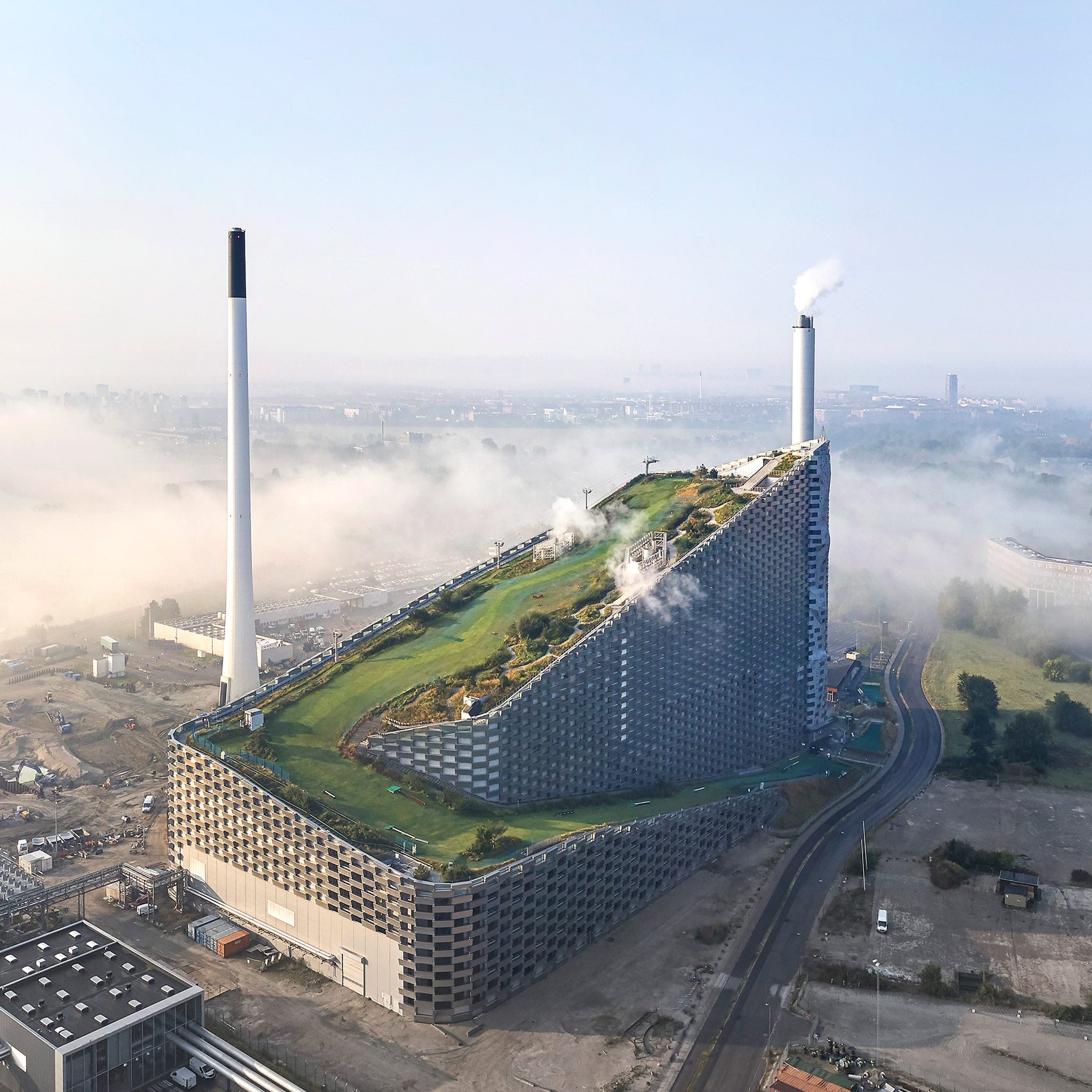The image showcases a surreal, AI-generated depiction of a massive industrial building in a bleak, urban environment. This futuristic structure is set along a typical highway, surrounded by smaller industrial buildings, empty fields, and rural areas. The most prominent feature of the building is its enormous grass ramp that starts at street level, loops around sharply, and ascends to the top, resembling a ski slope or a golf green. The base and sides of the building are lined with numerous windows, constructed from brown bricks or similar material, giving it a robust appearance. On each end of the building, two giant white smokestacks tower upwards, adding to its imposing presence. The surrounding landscape is desolate, with dirt, scattered vehicles, see-through bricks, and scattered patches of vegetation, heightening the sense that this is an artist's impression of a recycling plant or some imagined industrial complex. In the backdrop, a sprawling city is visible through a mist of brown, cloudy smoke, under a blue, yet hazy sky. The entire scene blends elements of industrialization with a touch of green, symbolizing a blend of nature and machinery in this fictional setting.